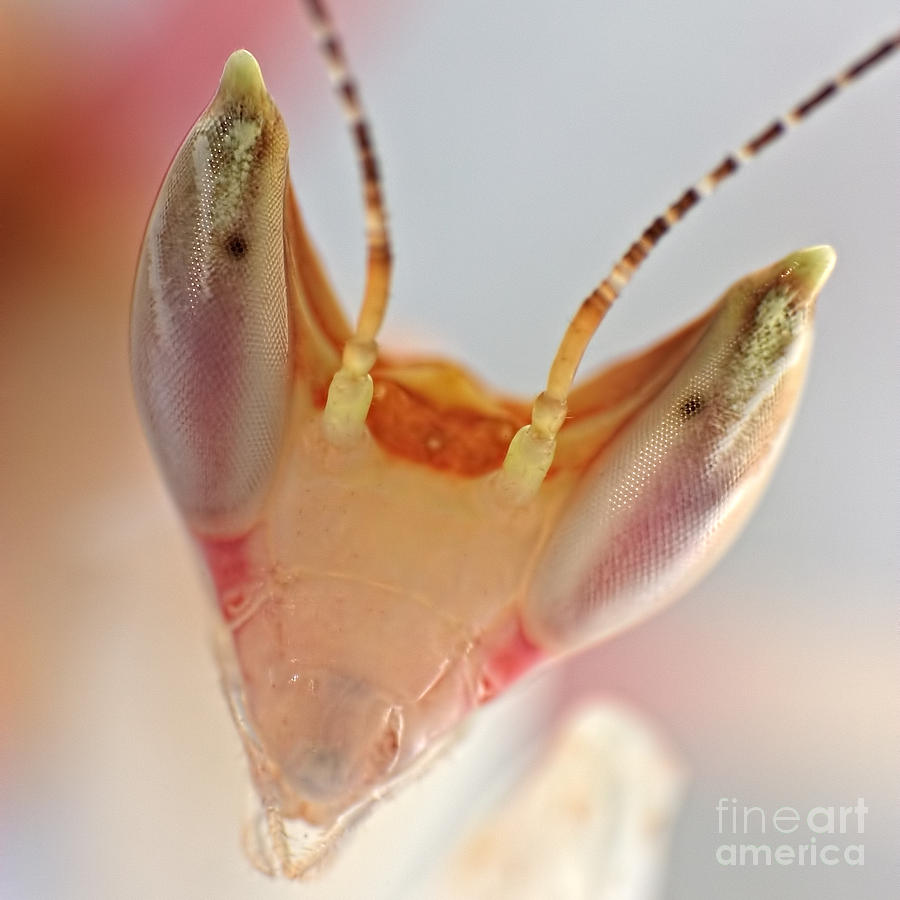This high-definition, close-up photograph from Fine Art America showcases the intricate head of an insect, likely a praying mantis. The magnified view allows you to see the detailed texture, akin to fish scales, and almost the individual cells of its two large, black eyes with oblong screening. The head is primarily light-colored with semi-translucent hues, featuring a palette of light pinks, yellows, and blush tones, accented with salmon pinky-orange and dull yellow shades. Two antennae, striped in shades of brown and white, extend from the base of the head. The bright, light image has a blurred background, drawing full attention to the fascinating details of the insect's head. The Fine Art America logo is visible in the bottom right corner.